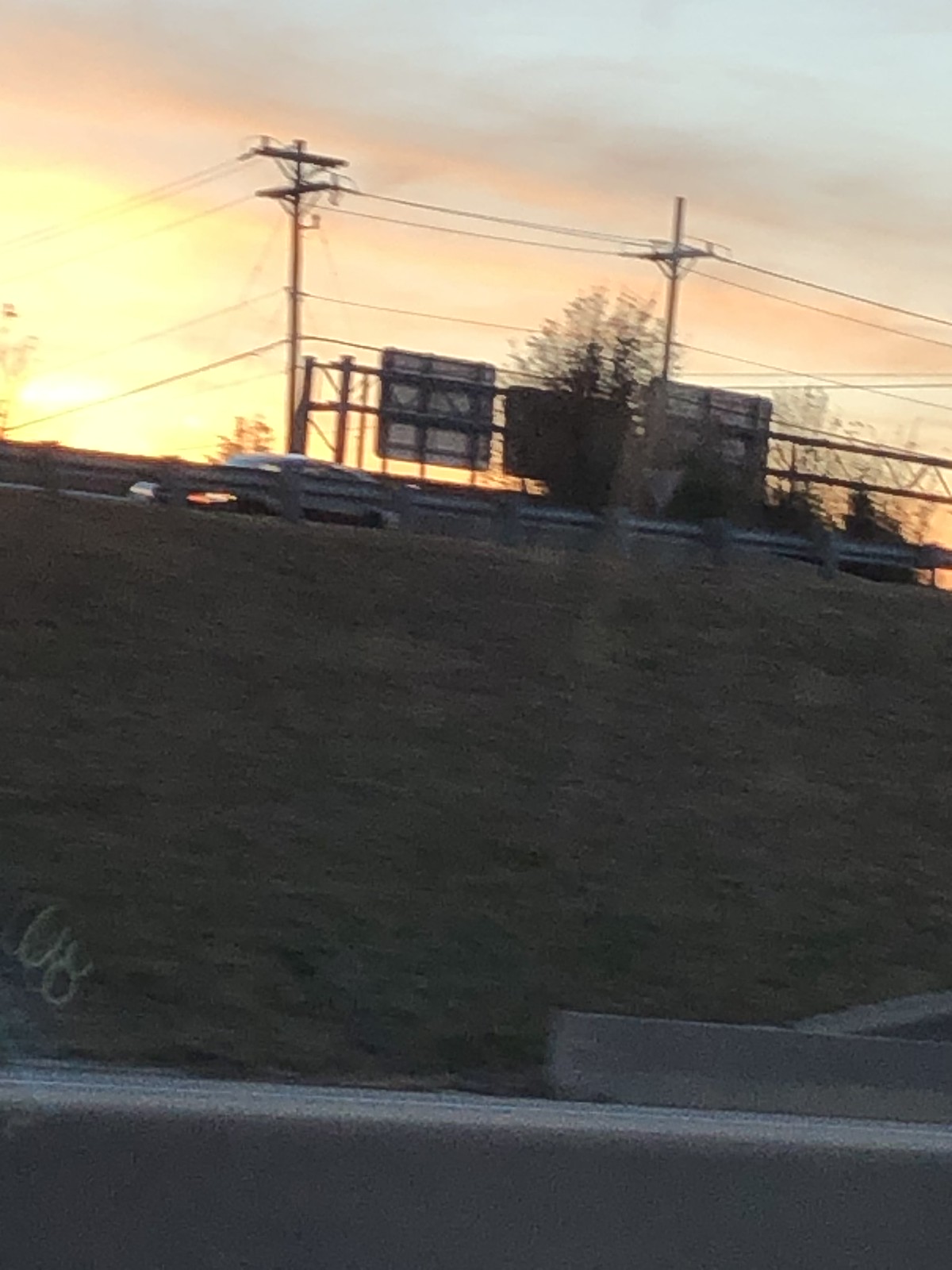This photograph captures a dynamic scene from the bottom of a grassy hill beside a road during sunset. The viewer's perspective appears to be from inside a car, suggested by paneling at the bottom of the image and possible window smears. The road ascends the hill, bordered by a metal guardrail, with a car travelling towards the left side of the image. Above the road, a series of road signs is visible, along with power lines stretching across the sky. The upper third of the image showcases a stunning sunset, with vibrant hues transitioning from bright yellow and white on the left, to orange, pinkish tones, and hints of blue and gray at the top. The car at the bottom remains in shadow, highlighting the contrast created by the descending sunlight.